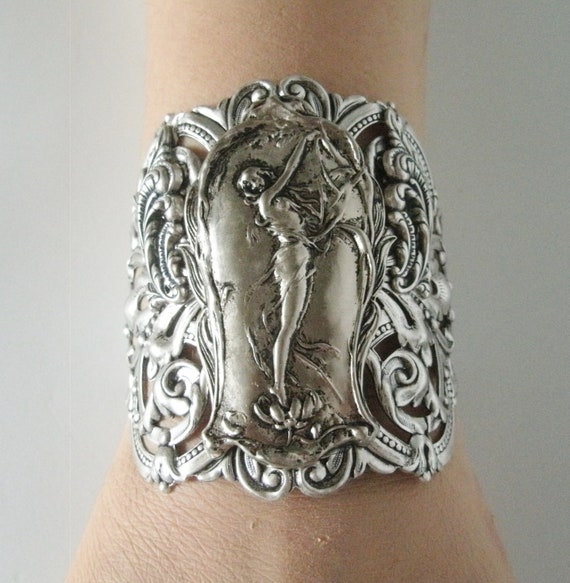The image features a light-skinned person's arm, prominently showcasing a distinctive bracelet that resembles a blend between a bracelet and a bangle, crafted from what appears to be silver. The intricately engraved bracelet includes floral accents and depicts a woman standing on a bed of flowers, which could be tulips. The woman is facing sideways but turns her head towards the viewer, her arms raised and extended ahead of her, and her head tipped back slightly. The background is a plain gray, likely representing wallpaper or flooring, highlighting the detailed craftsmanship of the bracelet. The skin near the bottom of the image has noticeable bumps.